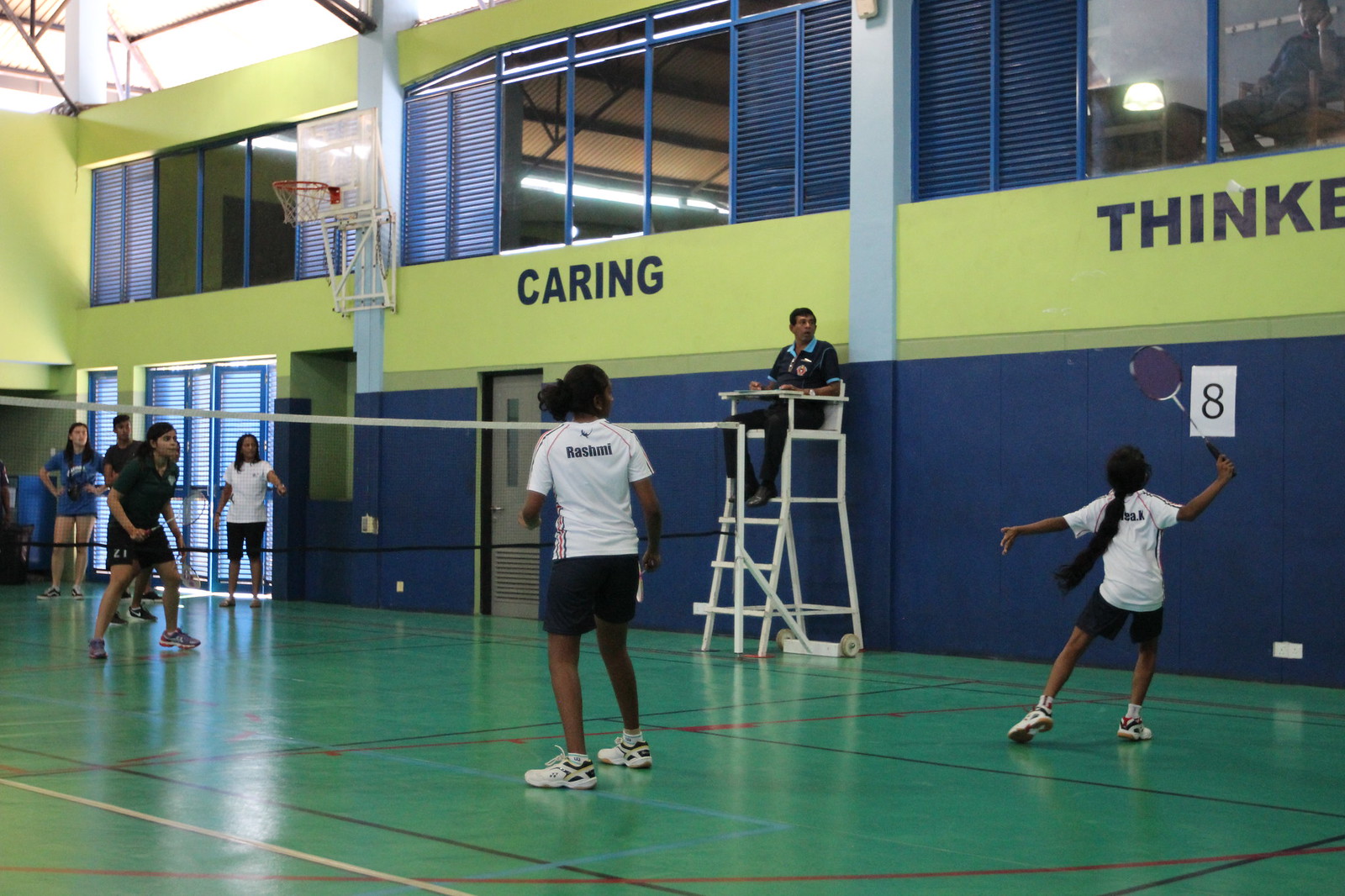In this horizontally-aligned rectangular image, an indoor badminton game is in progress. The gym's walls are decorated with blue on the bottom and yellow on top. The upper section features several windows; some are closed with horizontal blinds while others are without. The playing surface is a green court distinguished by blue and red lines, creating a colorful contrast. The viewer’s perspective captures the net stretching from the right edge to almost the left edge, where the pole is cut off by the image's frame. 

In the foreground, two female players in white shirts and black shorts dominate the scene. One player, with a long brown ponytail, has her arm raised, poised to hit the birdie. Next to the net, a referee clad in all black sits in a tall chair against the blue wall, overseeing the match. On the opposite side of the net, opposing players also wear black attire and appear ready to receive the shuttlecock. Spectators are casually scattered in the background, observing the game. Above, a basketball hoop is visible, hinting at the versatile use of the gym space. The words "Caring" and "Thinker" are noticeable on the wall, adding a thoughtful ambiance to the environment. The scene is lively, with various hues including green, red, dark blue, and lime green adding vibrancy, indicating the match is taking place in the middle of the day.